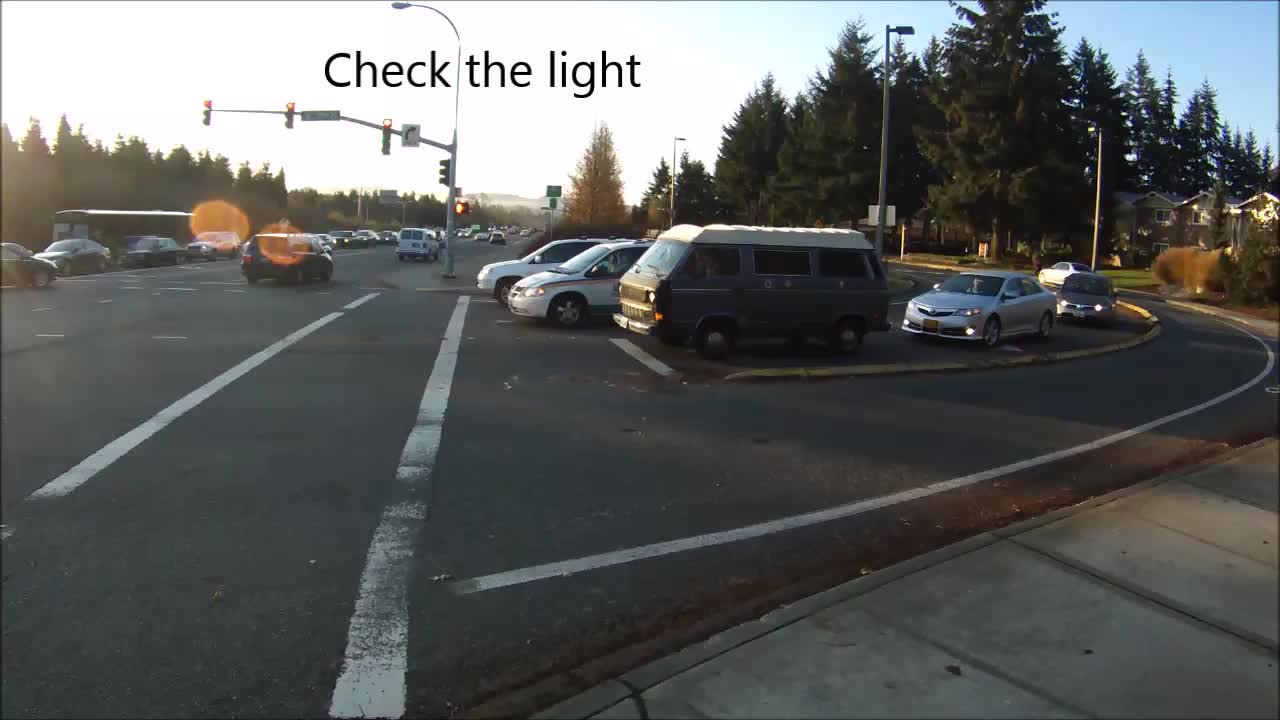The photo captures a bustling intersection where two roads converge under a red traffic light. The primary road runs straight through the scene, while the secondary road curves off to the right, vanishing into a dense cluster of trees. These trees obscure several homes in the background, lending the area a secluded, suburban feel. Dominating the foreground is a light pole adorned with multiple red stoplights, dictating the flow of vehicles. A variety of cars, including a classic Volkswagen camping bus, several vans, SUVs, and other vehicles, are queued at the light, poised to join the main straight road. This straight road appears busy, with a line of cars stretching into the distant horizon, framed by additional greenery. The overall atmosphere is one of a typical day at a busy suburban junction, where modern vehicles contrast with the tranquility of surrounding nature.